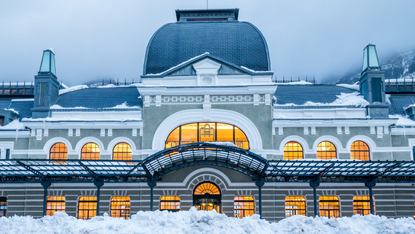The image depicts a grand, ornate building, potentially reminiscent of Russian architecture, set against a cloudy, grey sky. The structure features a striking dark blue, oval-shaped roof and a lower-level roof of the same blue hue, both dusted with snow. The building itself is gray with white trim and boasts numerous beautifully designed arched windows. The central part of the building includes a large rounded window, flanked on each side by additional arched windows, making for a total of seven arches on one level, with an additional arched doorway centrally located. Below these, eight square windows and a single arched window are visible. Warm, orange-yellow lights glow from within, contrasting with the exterior's chilly, wintry scene. Snow blankets the ground and the roof, enhancing the wintery ambience, and in the background, majestic mountains complete the picturesque setting.